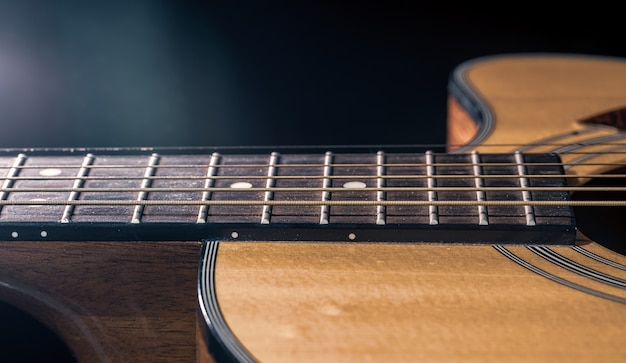The image features a close-up of an acoustic guitar lying flat on a polished wooden table. The guitar, which is a light tan color, is seen from above, showcasing a section of its body and the lower part of its neck. The neck, adorned with frets and six strings, extends from the left side of the image towards the right. Notably, the guitar includes a cutout allowing access to higher notes and the sound hole surrounded by decorative gray and white lines. The dark background contrasts with the light-colored guitar, drawing focus to its details. There are no humans or text present in the scene, emphasizing the guitar itself.